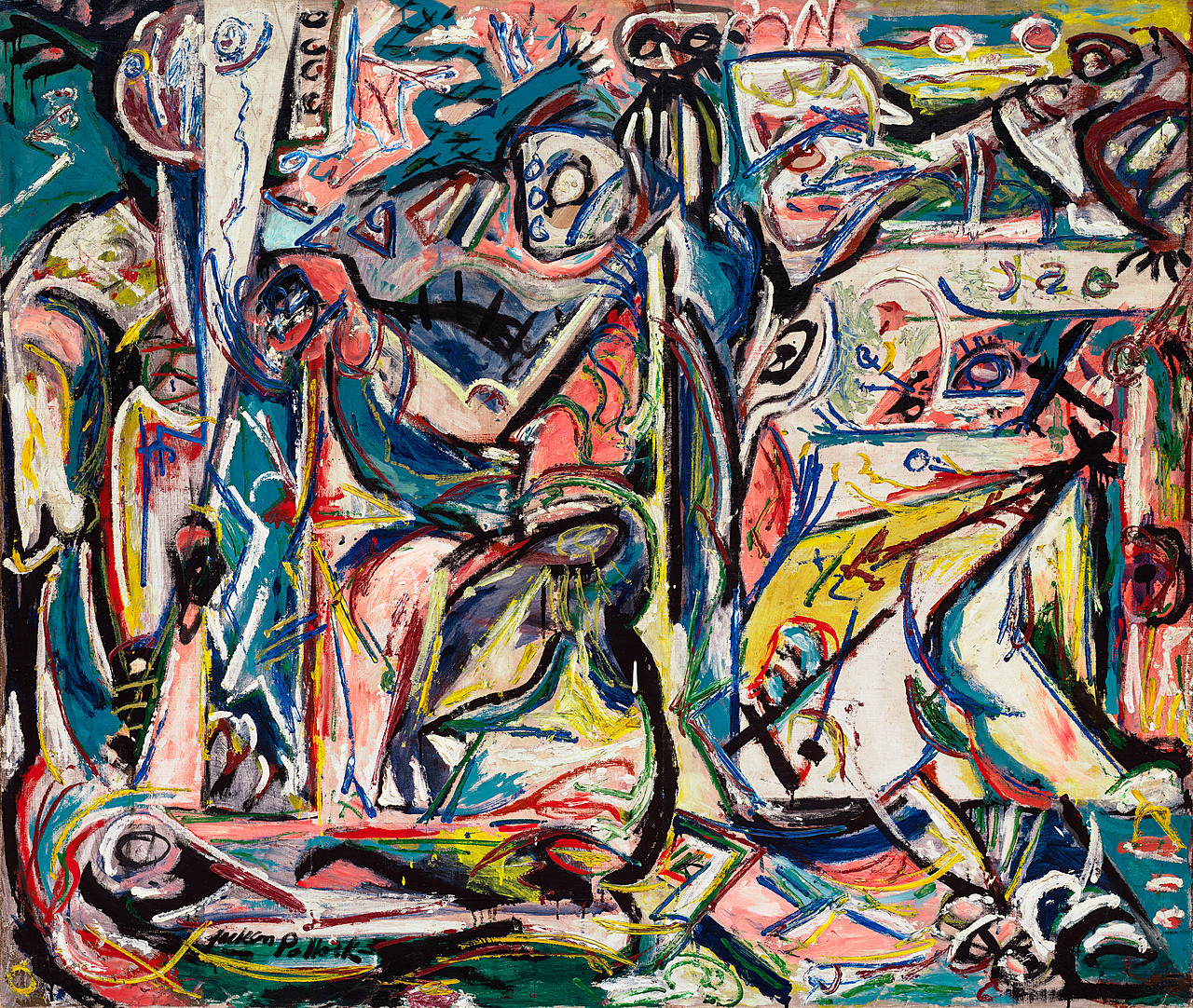This vibrant and chaotic abstract painting features a dynamic interplay of colors and geometric shapes, creating a visually stimulating composition. Predominantly set against a blue background, the artwork is accented with vibrant hues of pink, orange, red, yellow, and touches of beige, representing nearly every color of the rainbow. The canvas is filled with an array of overlapping shapes such as circles, various triangles, and squares, blurring the boundaries between them and creating a sense of depth and complexity. At the bottom right corner, what seems to resemble a table can be discerned. Scattered throughout the piece are elements that evoke facial features—eyes with prominent eyelashes, noses, and mouths—suggesting hidden figures, some appearing to bend over, others seemingly peering out at the viewer. Notably, at the very top of the design, there is a form that hints at an alien-like creature with an oval body and a head with large eyes. The artist's signature, "Pa House," is visible at the bottom left corner, anchoring this mesmerizing and enigmatic composition.